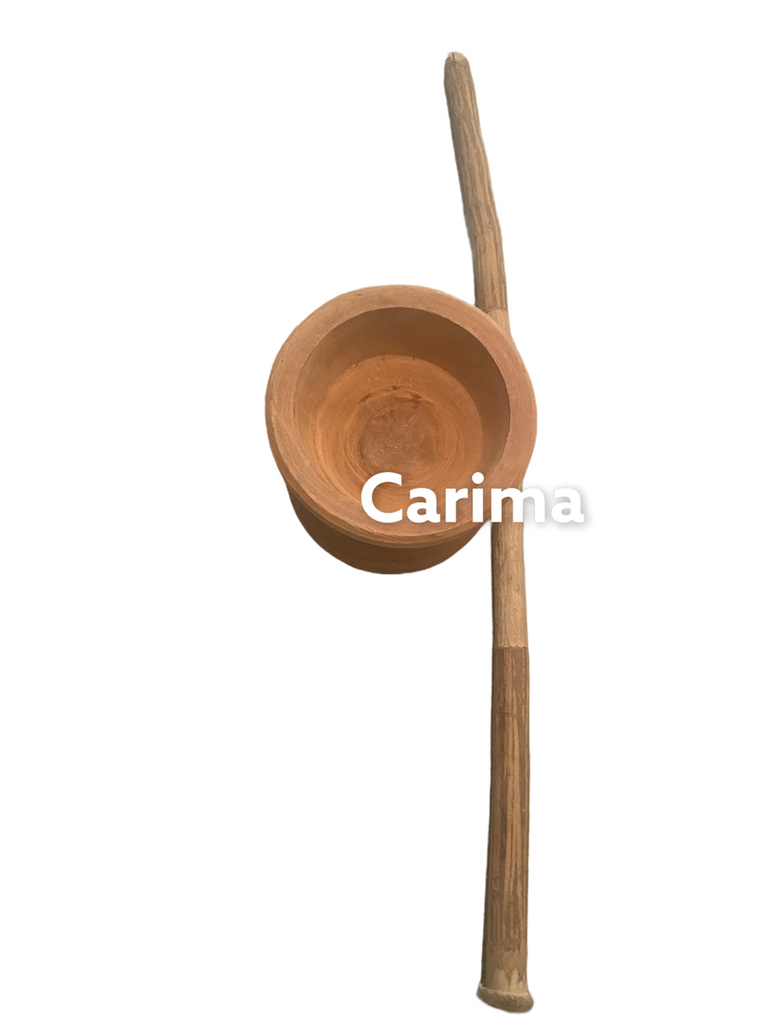The image depicts a light-colored wooden staff with a slightly bent top towards the left. This staff appears largely unaltered except for a slightly wider section near its midsection, which may have been carved for subtle design features. The base of the staff, which touches the ground, is more rounded. Beside it lies a small clay bowl, brown in color. The scene is shot from a top view, with the text "Karima" spelled out in white ink across the bowl and part of the staff.